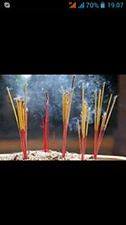The image, an extremely low-quality screenshot from a mobile phone, showcases five bundles of sticks—likely either sparklers or incense sticks—stuck into the ground and emitting smoke. The overall image is quite small with significant black bars at the top and bottom, indicating it was captured in a horizontal format. The screen displays phone icons, including battery life at 70%, a Skype notification, and the time showing as 19:07. The sticks appear red with golden tops and are releasing curling, misty, gray smoke. Despite the blurred quality, the arrangement and characteristics of the sticks suggest a setting possibly related to some form of ritual or celebration.